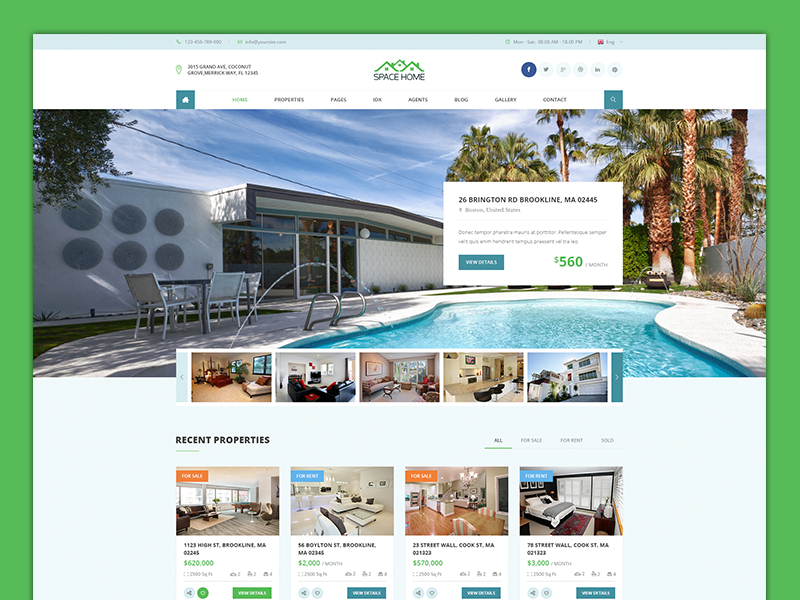This image features a web page with a clean white background, framed by a green-colored backdrop visible along its edges. At the top of the web page, a sleek gray bar spans across the width, hosting black text that includes navigation buttons for language settings, menu items, emails, and contact numbers. On the left side of this gray bar, an email address and a phone number are prominently displayed.

Directly beneath the gray bar, a large rectangular section showcases the company’s logo, which depicts a set of houses with green roofs, accompanied by the text "Space Home" in bold black font. Adjacent to this are icons for various social media platforms including Facebook and Twitter.

Below this logo section lies a navigation bar with buttons labeled in black text, directing users to different sections of the website: Home, Properties, Pages, Agents, Blog, Gallery, and Contact. To the far right of this bar is a prominent blue search button.

Taking center stage on the page is a large, vibrant rectangular photo featuring a picturesque backyard swimming pool surrounded by tropical trees under a bright blue sky. Beneath this main image, there are additional smaller photos showcasing the interiors of the property, alongside images of other hotels and accommodation options, illustrating various places to stay.